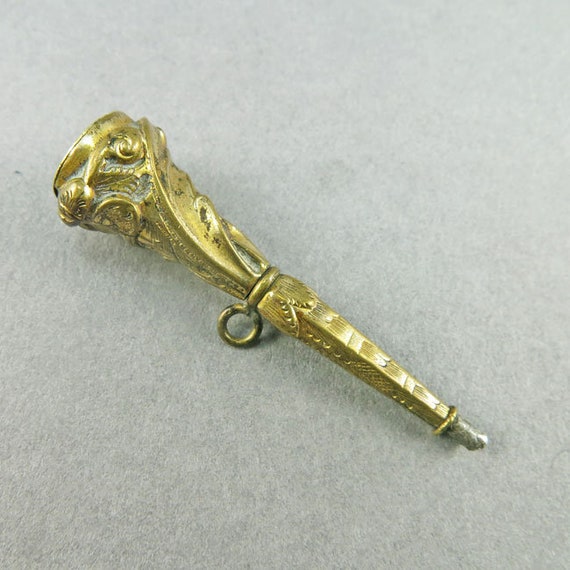The image depicts a vintage, gold-colored item laying on a flat, white, possibly microfiber background. The object is likely a pendant, shaped somewhat like a torch or elongated nail, with a wider top on the left that narrows down to a slender body on the right. Intricate leaf-like or fine designs embellish its surface. In the middle of the object, there's a piece that forms a loop, suggesting it could be strung on a necklace, supporting the pendant theory. A band encircles the bottom, accompanied by a small, possibly silver element hanging at the tip. Despite its detailed craftsmanship, the exact purpose of the item remains unclear.